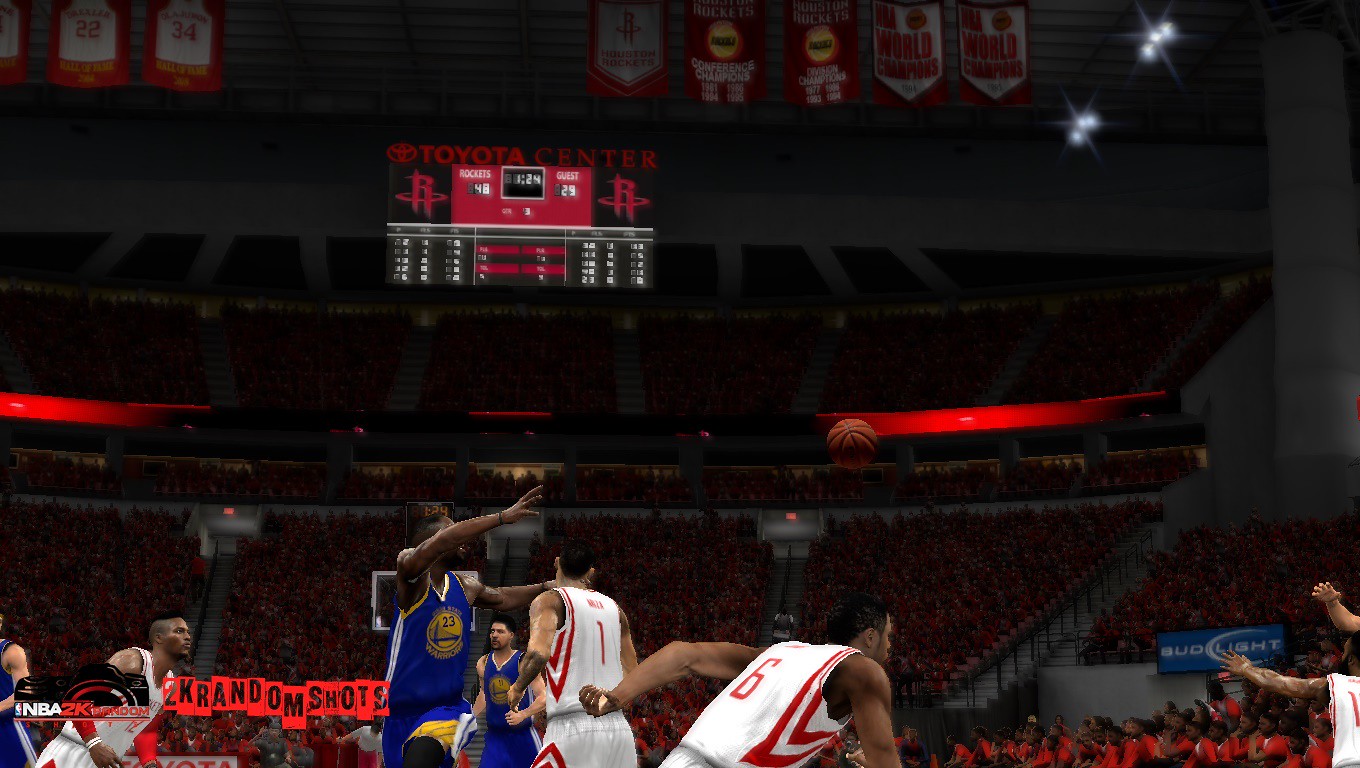The image is a detailed still from the video game NBA 2K, capturing a realistic depiction of a basketball game. The game is set in an arena prominently displaying "Toyota Center" above a scoreboard. The scoreboard indicates that the Rockets lead with 48 points over the Guest team's 29 points, with 1:24 remaining in the game. Two teams are playing: one team is in white jerseys with red trim, and the other team is in blue jerseys with a golden insignia resembling the Golden Gate Bridge.

In the foreground, a player in a blue jersey is reaching out to pass the basketball to a player off-screen while opponents in white jerseys attempt to block him. Another two players in white jerseys are located to the left, seemingly disengaged from the action. The crowd in the background, uniformly dressed in red, enhances the vibrant and immersive atmosphere of the simulated arena. Advertisements for Monster Energy Drink flank the scoreboard, and various jersey and championship banners hang from the rafters. A watermark reading "NBA 2K Fandom" and "2K Random Shots" is visible in the lower left-hand corner, indicating the game's branding.